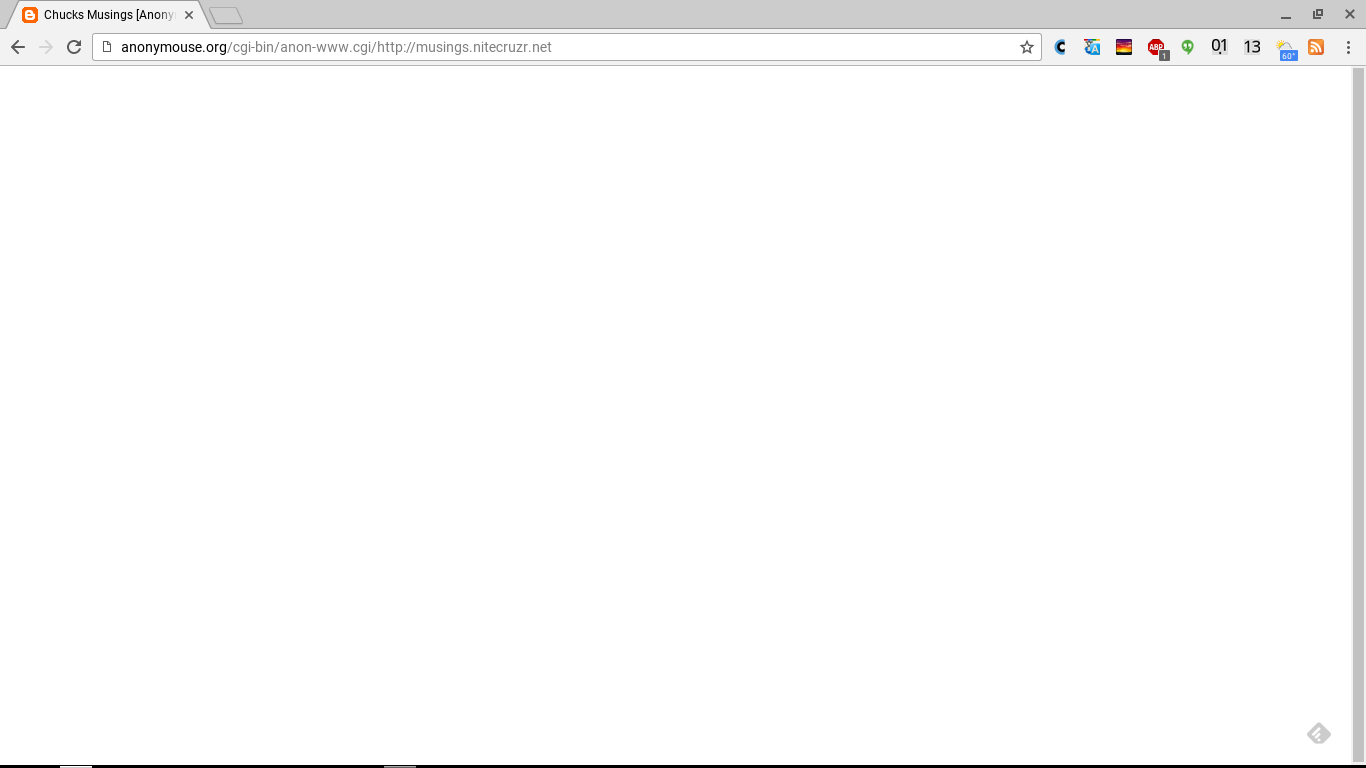A screenshot of a website displayed in portrait orientation, resembling the dimensions typically seen on a desktop or laptop screen. The image lacks a defined border but features a horizontal grey or black bar at the bottom. At the top, a long, horizontal grey header displays an open tab labeled "Chuck's Musings," though the full title is cut off. Beneath the header, a grey bar houses navigation elements, including a back arrow, a greyed-out forward arrow, a refresh button, and a URL box showing the address "annoymouse.org" followed by grey subheadings. A star icon and various other icons are positioned to the right of the URL box.

The main content area below the navigation bar is occupied by a white rectangular box, which appears to be landscape in orientation. This box is devoid of text or other content, suggesting a possible broken link or an empty webpage. At the bottom of the screen, there's a diamond-shaped grey watermark featuring two shades: lighter grey on the left and darker grey on the right. On the right edge of the screenshot, a vertical grey bar functions as a toggle or scroll bar, but offers no additional details.